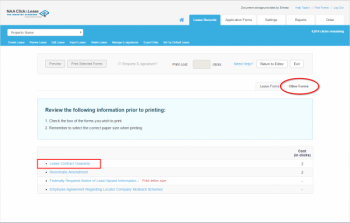A small screen capture displays a portion of a computer interface, either from a webpage or an application. At the top is a grey navigation bar listing an unreadable company name, accompanied by multiple menu choices to its right. Overlapping this grey bar is another grey section presenting several tabs for navigation. The nearly centered first tab is highlighted, followed by four additional tabs extending towards the right side of the screen.

Beneath the tabs, a dark blue bar contains a text entry box, designed for inputting selections, along with additional words scattered across the dark blue background. Below this, there are several unhighlighted buttons providing different options.

The main interface area is predominantly white, featuring a couple of option buttons, one of which is circled in red. Further down, highlighted in a greenish-blue box, is a message instructing users to review specific information before proceeding with pricing, accompanied by two selectable options.

At the bottom of the screen are a few selection boxes containing lists accompanied by notes or names. The first item in one of these lists is distinctly marked with a red box.